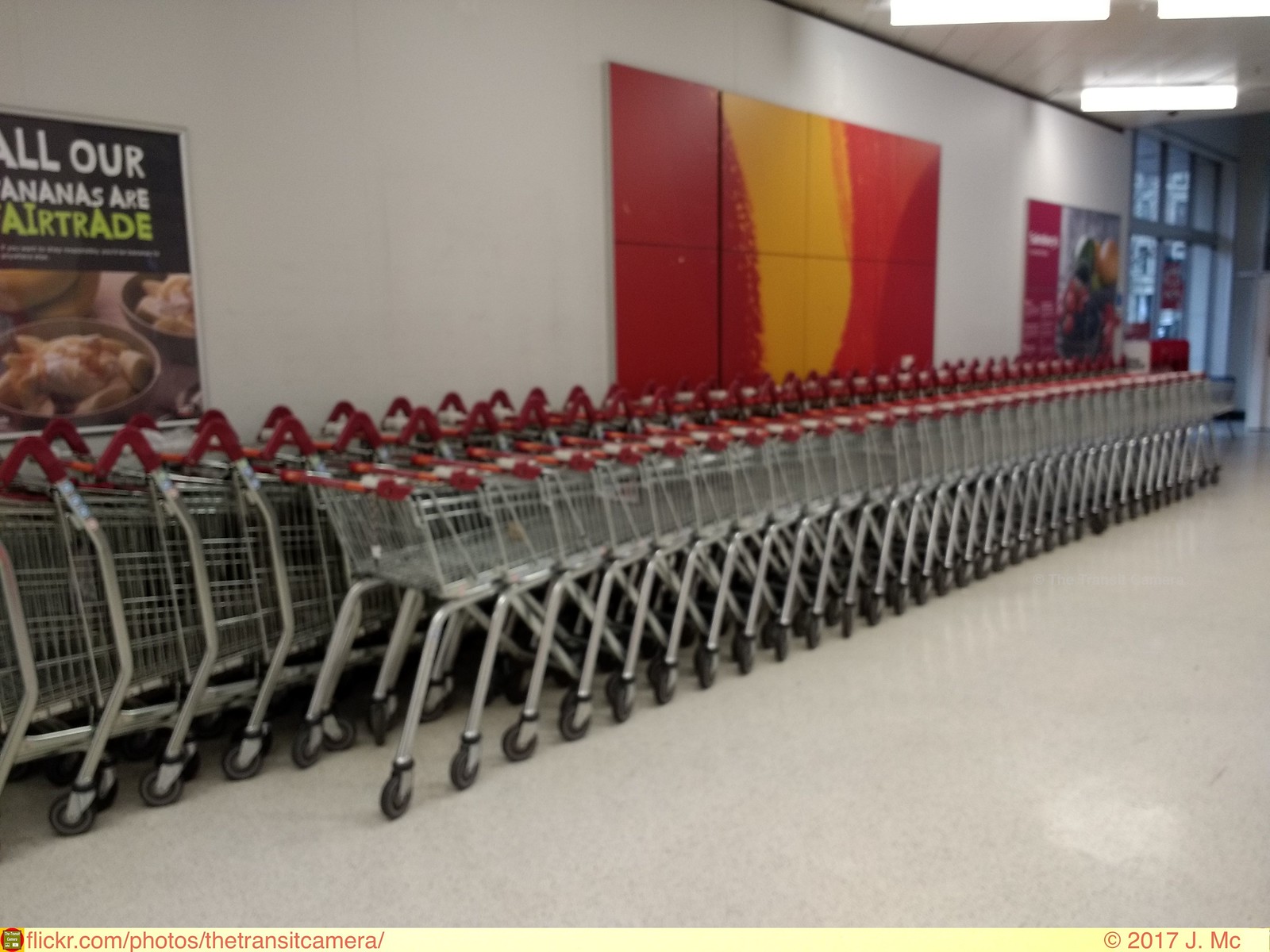The image is a slightly grainy, low-quality color snapshot taken inside a supermarket. It features a line of over 20 metal shopping carts with red handles, positioned in a diagonal row against a white wall. The shopping carts range in size, with larger ones closer to the wall and smaller, miniature ones further away. 

On the left-hand side of the image, there is a poster partially visible at the top, which reads "All our bananas are Fair Trade" with a picture of bananas. Additionally, the wall displays other indistinct advertisements. In the center of the image, there's a prominent red and yellow abstract design or mural. At the far end of the line of shopping carts, a door is visible with sunlight streaming through it.

The floor is beige and the top-right corner of the image shows fluorescent lighting hanging from the ceiling. The bottom portion of the image has a yellow stripe containing text: "flickr.com/photos/thetransitcamera/  © 2017 JMC."